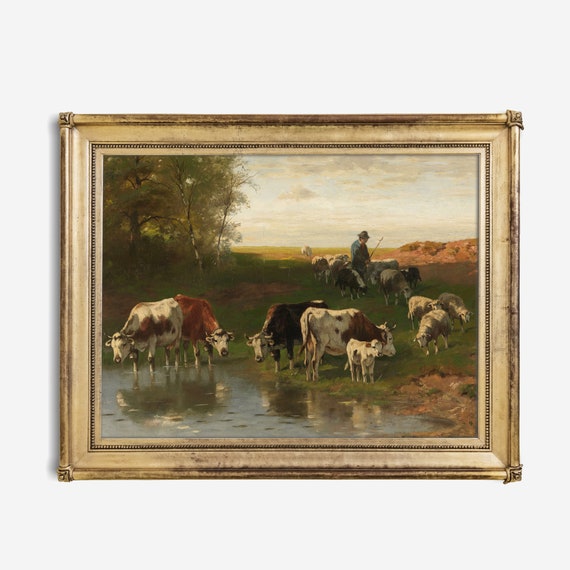This is a color photograph of an oil painting, set in a somewhat weathered yet detailed gold frame, hanging on a plain white wall. The painting depicts a serene farmland scene, where several cows, in shades of brown, camel, and black, are gathered at the base of a pond, drinking water. Their reflections are visible on the pond's surface. A cow with a calf stands to the left, looking towards a group of sheep approaching the watering hole. In the background, a farmer dressed in blue with a blue hat is seen guiding the sheep. Beyond the grazing animals, green trees and bushes can be observed, while white, hazel-tinged clouds drift across a light blue sky, suggesting a calm daytime setting. The frame's simple golden design with corner detailing complements the pastoral tranquility of the scene.